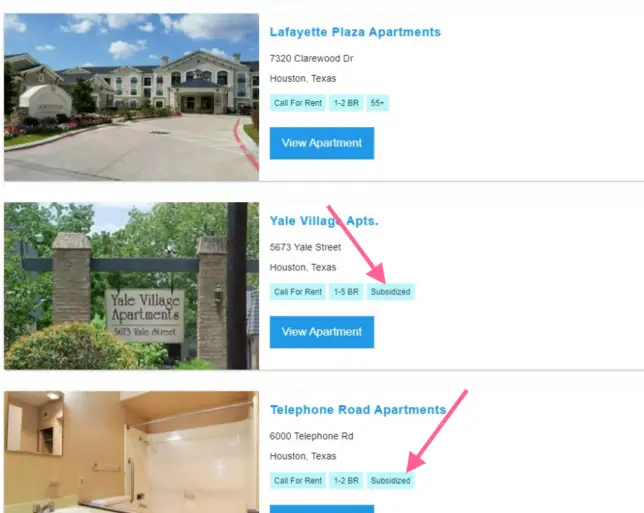This image is a screenshot from a website, divided into three vertical panels. 

The first panel on the left features a photograph of an apartment complex. The image depicts a large white building under a blue sky dotted with white clouds. A driveway leads to the building, and in the foreground, there’s a sign surrounded by flowers and grass. To the right of the image, blue text reads "Lafayette Plaza Apartments," followed by smaller black text stating "7320 Clairwood Drive, Houston, Texas." Additional information indicates the property offers one to two-bedroom units for individuals aged 55 and older, with a prompt to "Call for rent." A blue banner with white text invites viewers to "View apartment."

The second panel captures an outdoor scene with a blue sky and some cloud cover. The view includes trees and two pillars connected by a metal bar, which supports a hanging sign that reads "Yale Village Apartments." Below, black text provides the address "5673 Yale Street, Houston, Texas," along with a note that these apartments offer one to five-bedroom, subsidized units. A red arrow highlights the word "subsidized," and a blue, clickable banner with black text instructs viewers to "View apartment." 

The third panel depicts an interior shot of a bathroom, showcasing a wall with a mirror, a sink, and a bathtub. Accompanying the image, text reads "Telephone Road Apartments," followed by the address "6000 Telephone Road, Houston, Texas." The apartments feature one to two-bedroom, subsidized units, with a red arrow pointing at the term "subsidized."